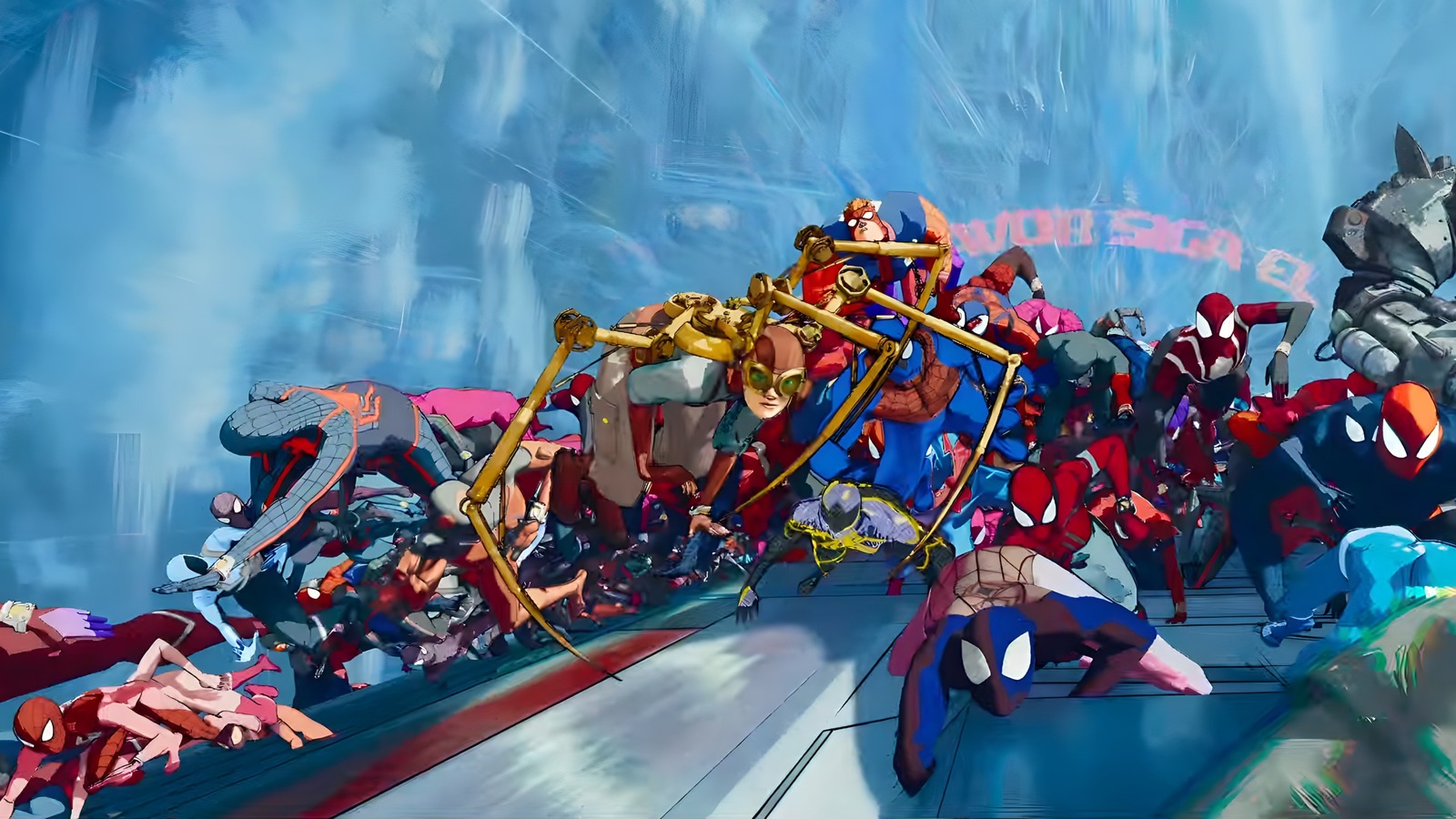The image depicts a vibrant, chaotic scene of various Spider-Man-like figures, rendered in a detailed, cartoon style with a predominantly blue and colorful palette. Among them, several Spider-Man variants showcase unique costumes, including one with blue and purple attire, another gray with orange spider emblems and stripes, and a third with an orange head and blue body. The backdrop features a pink text banner across the top, reading "Saga E.L." faintly, and a blue background interspersed with abstract art elements. The characters appear to be either scaling or falling from a building, with a metallic, gold spider perched atop the crowd, invoking a blend of urgency and action, suggesting a scene of either combat or rescue in the midst of this tangled, dynamic tableau.